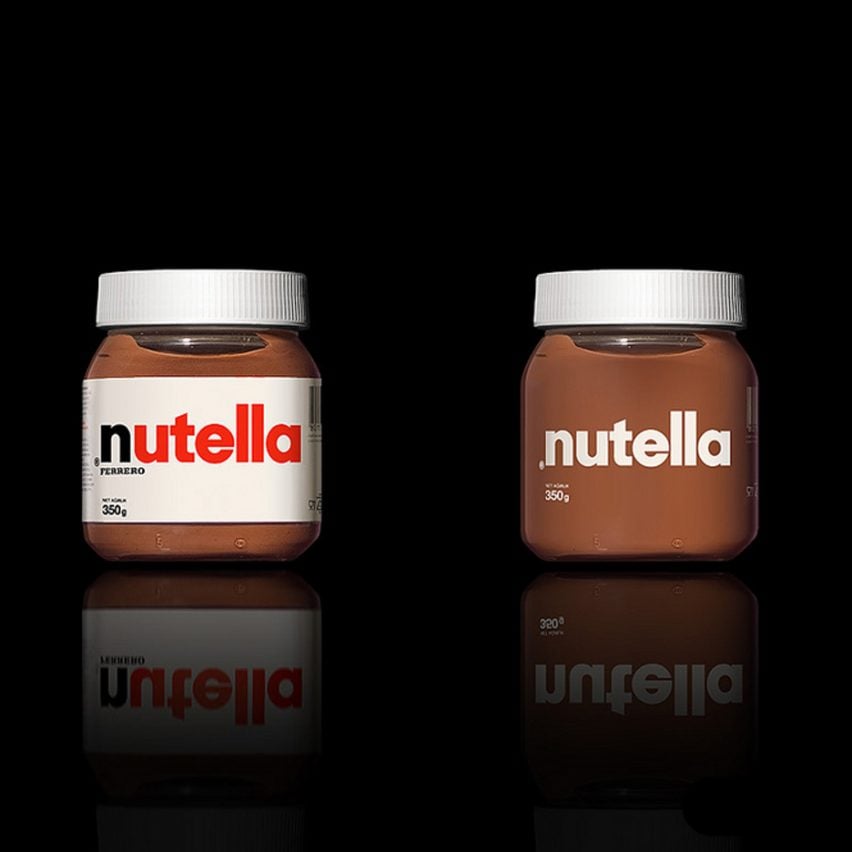The image is a square photograph displaying two jars of Nutella against a black background. The surface they are resting on is reflective, mirroring the jars, which creates an elegant, almost advertised look. On the left is a typical Nutella jar featuring a white perforated lid and a white label. The label has "Nutella" with the 'N' in black and the rest of the word in red, followed by "Ferrero" in black font, indicating the brand. The jar contains the familiar brown Nutella spread. Beside it, on the right, is a more minimalist Nutella jar. It also has a white perforated lid but lacks the traditional label, instead, displaying "Nutella" in lowercase white font directly on the clear jar, which allows the brown spread to be visible. Both jars are marked with a weight of 350 grams. The lighting highlights the jars, emphasizing their features in the clean, simple composition.